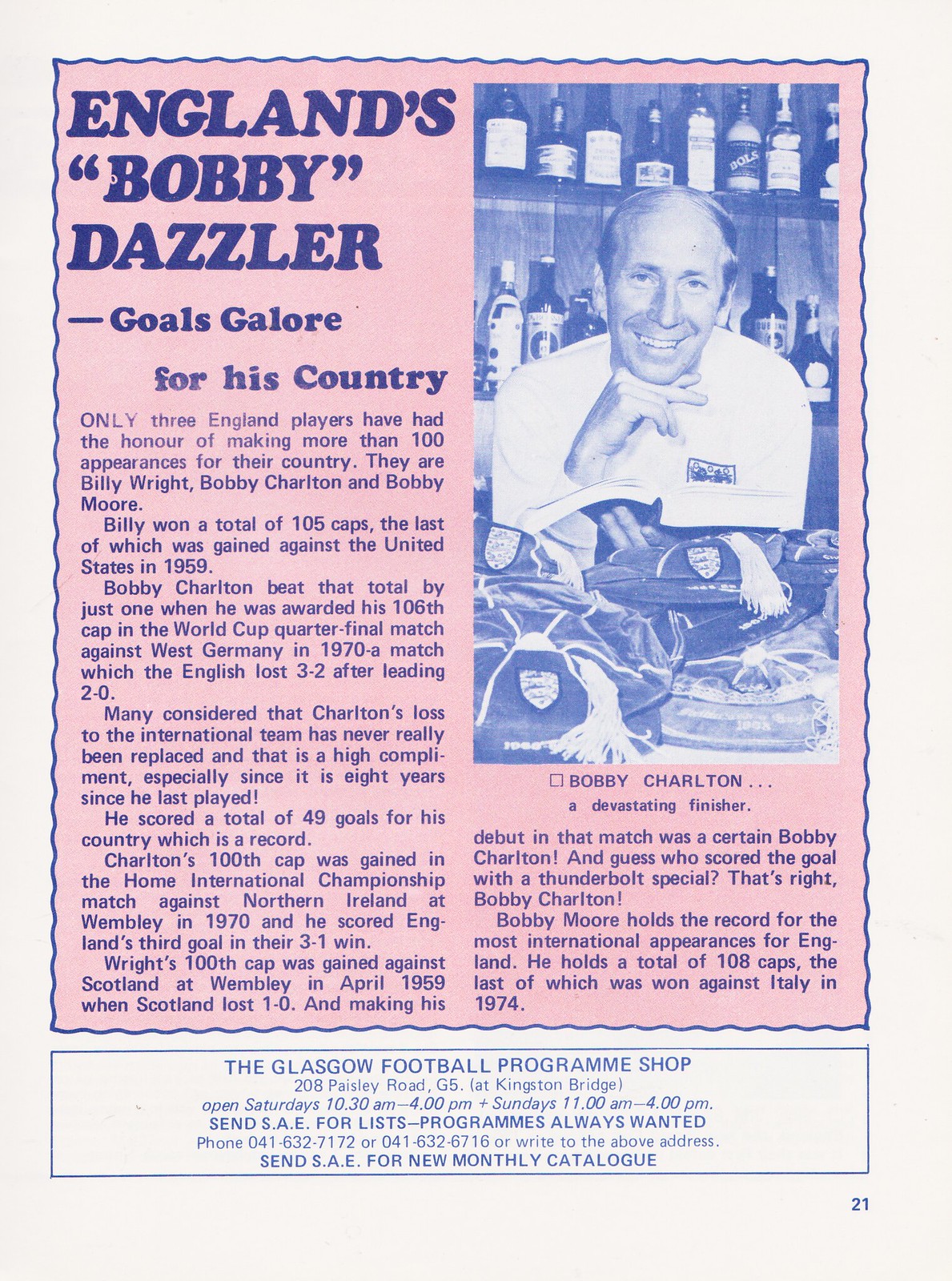This is a detailed description of page 21 from a Scottish football program, likely from a magazine related to soccer matches. The page features a predominantly pink background and is titled "England's Bobby Dazzler: Goals Galore for His Country." The central focus is an article about the legendary English footballer Bobby Charlton, known for his significant contributions to his national team. 

The article sits in a two-column layout, with a photograph accompanying it on the right-hand side. The photo depicts Bobby Charlton, a clean-shaven, balding gentleman in his 40s or 50s, sporting a white shirt and a big smile. He is posed with his hand under his chin, set against a backdrop of shelves stocked with various liquor bottles, suggesting a possible setting in a liquor store.

The article highlights Charlton's remarkable career, noting that he is one of three England players to have earned over a hundred caps for representing his country, alongside Billy Wright and Bobby Moore. Specific achievements mentioned include his 106th cap during the 1970 World Cup quarterfinal against West Germany and his 100th cap in the Home International Championship against Northern Ireland at Wembley in 1970. The narrative acknowledges his record of 49 goals for England and underscores his irreplaceable impact on the team.

At the bottom of the page, framed by a thin blue border, are details about the Glasgow Football Program Shop located at Kingston Bridge, 208 Paisley Road. It mentions the shop's operating hours on weekends, the process for obtaining a program, and the availability of a monthly catalog via a self-addressed stamped envelope.

This snapshot captures both the enduring legacy of Bobby Charlton and the cultural significance of football memorabilia in the UK.